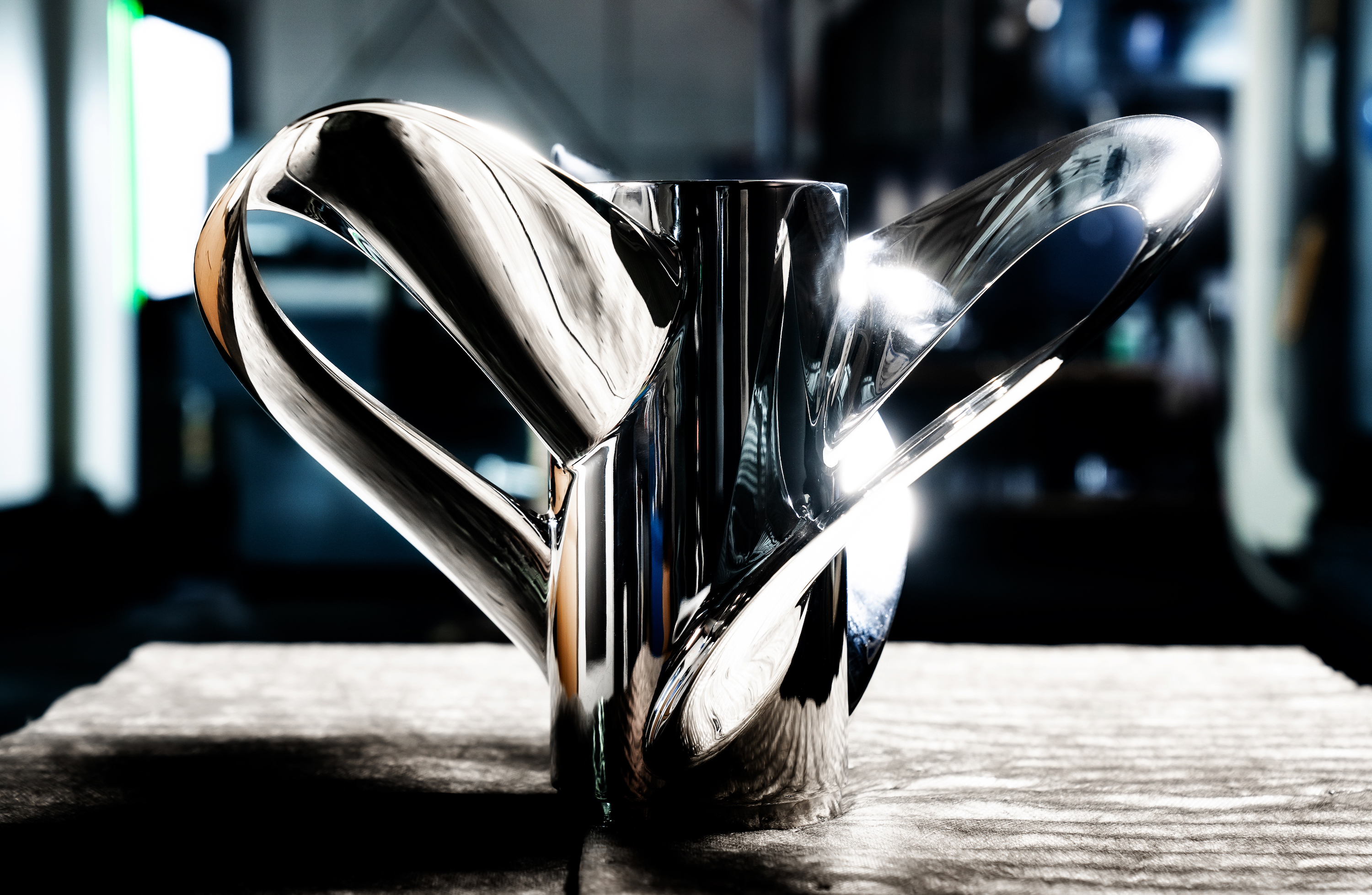The image is a Surrealist depiction of a peculiar, angular vase or carafe made of polished silver with intricate, overlapping curved handles. The object is central in the image, placed on a gray wooden table with light cascading from the right side, casting minimal yet distinct reflections. These reflections, although not very pronounced, reveal a green and white striped blanket and fragmented, colorful strips, possibly hinting at figures. The background remains distinctly blurry with an apparent white column on the right and a neon green strip on the left, adding to the surreal ambiance. The vessel is tall, its metallic surface lustrous, and its form enigmatic, suggesting various utilities from serving drinks to holding plants. Despite the indistinct surroundings, the object's shiny, rich sterling silver appearance stands out strikingly.